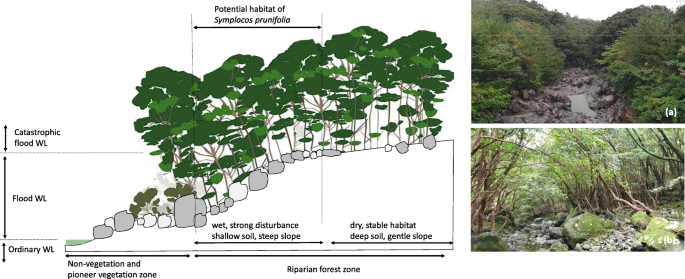The image depicts a detailed nature diagram primarily focused on illustrating different types of habitats and flood zones within a sloped, forested rocky area. On the left side, the diagram includes labels indicating "catastrophic flood WL," "flood WL," and "ordinary WL," with a black arrow marked as the "potential habitat of Simplocos pronifolia" along the slope. The slope starts low on the left and rises towards the middle-right, illustrating the gradient. At the bottom of the diagram, various habitat zones are labeled, including "non-vegetative," "pioneer vegetative zone," "wet strong deservance," "shallow slopes," "deep zone," "dry stable habitat," "deep soil," and "gentle slope."

On the right side of the image, there are two additional photographs identified as habitat areas. The top photo, labeled "A," showcases a lush forest area with tall green trees flanking a small stream. The bottom photo, labeled "B," shows a rocky terrain with a river flowing through it, with trees growing amidst the rocks and creating a canopy above the river. Both images collectively highlight the riparian and rocky forest zones, emphasizing the diverse ecological niches within the flood-affected forest landscape.